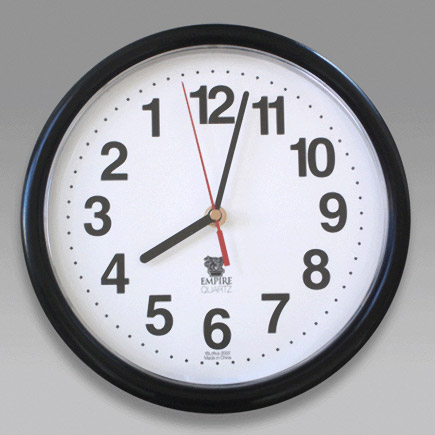This image showcases a color photograph of a round clock placed against a grey surface, which exhibits a gradient from darker at the top to slightly lighter at the bottom, with a small shadow visible beneath the clock. The clock features a black round edge and black numerals, arranged in an unconventional anti-clockwise sequence, where '1' appears at the position typically occupied by '11', '2' replaces '10', and so forth. The clock's black hour and minute hands indicate the time as approximately 4:55, while a thinner red second hand points between '12' and '1'. A subtle line of thin dots is visible just outside the black numerals, adding to the clock's detailing. A black logo with unreadable text is located just beneath the hands, and smaller writing is present below the numeral '6' at the bottom.